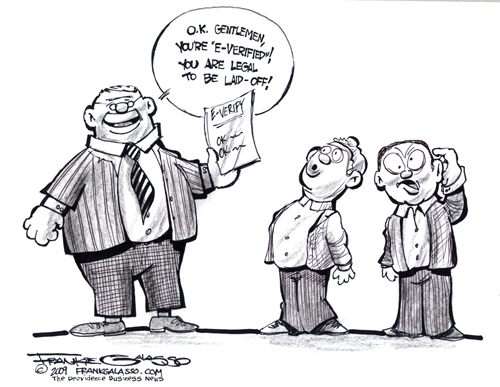This is a black and white cartoon, seemingly old-fashioned, drawn in pencil, and created by Frank Galasso in 2009 for The Providence Business News. On the left side, there is a heavyset, older man with a wide head and wire-rim glasses that bow outward to fit his head. He is smiling, wearing a suit coat with pinstripes, a collared shirt, a striped tie, and checkered pants. He holds a piece of paper in his left hand that says, "E-Verify, OK, OK," followed by some illegible scribbles. A speech balloon above him reads, "OK, gentlemen, you're E-Verified! You are legal to be laid off!" To his left, two shorter men appear shocked. One has his mouth shaped like an "O" in surprise, while the other has a confused expression with a finger next to his ear, as if signaling disbelief. The image is signed at the bottom left with "Frank Galasso, 2009," and "frankgalasso.com."